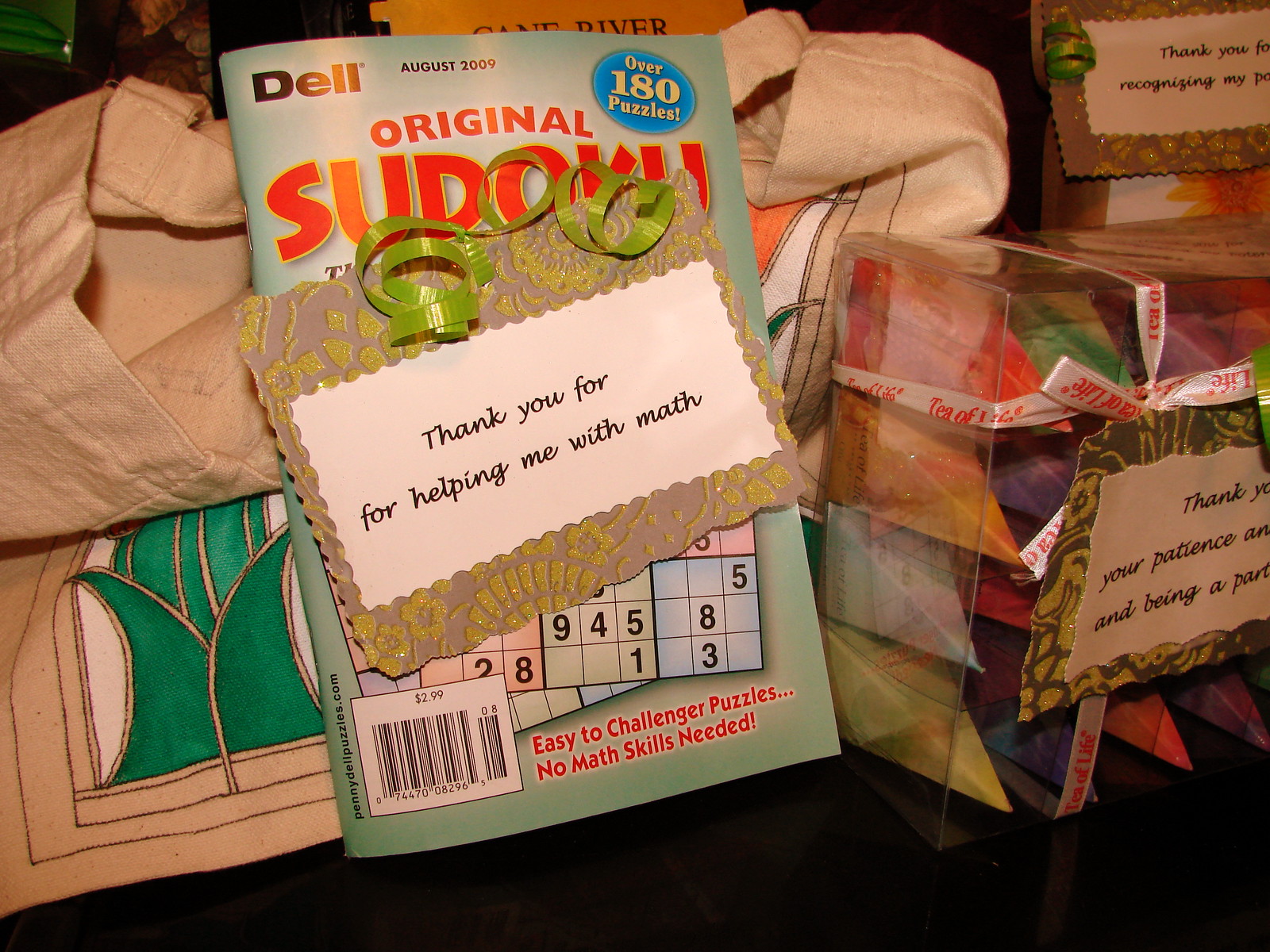The photograph depicts a cluttered shelf or table surface filled with various items and thank you notes. On the left side, a tan-colored tote bag or blanket, adorned with a green leaf, supports a green-covered Sudoku book from August 2009, labeled with "Dell" and "over 180 puzzles." Attached to this book is a glittery piece of paper with a white note, reading "thank you for helping me with math," tied with a green ribbon. To the right, there is a plastic box containing colorful pyramids, which could be bath bombs, accompanied by a note partly visible and reading "thank you for recognizing my potential" amidst other cut-off text. Scattered on the shelf or table are additional items, some appearing to be gifts or trinkets, each with individual thank-you notes attached. The scene collectively portrays a collection of gratitude tokens, each annotated with personal messages of thanks and decorated with various ribbons and tags.